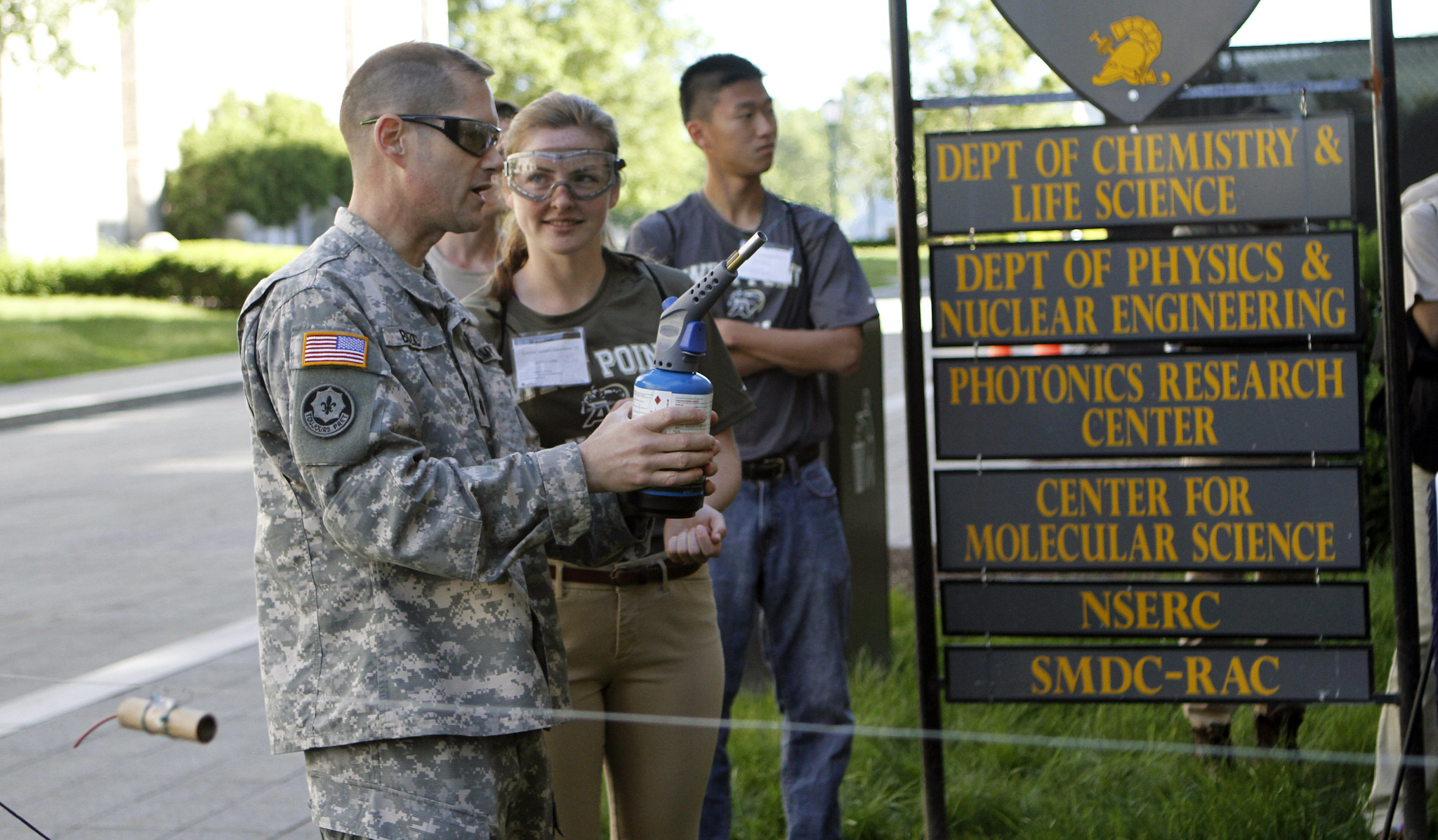The image depicts a daytime scene with a soldier and several other people standing near a series of informational signs. The soldier, dressed in a digital urban camouflage uniform with an American flag patch on his shoulder, has short hair and wears black-framed sunglasses. He is holding a blue canister with a white label using both hands, which seems to have a metallic protrusion at the top. Next to him stands a woman with blonde hair, wearing white chemistry lab goggles, a dark gray shirt—or possibly a West Point t-shirt—and light brown pants with a brown belt. 

To the left of the group are multiple rectangular signs with yellow writing, detailing various academic departments and research centers: Department of Chemistry and Life Science, Department of Physics and Nuclear Engineering, Photonics Research Center, and Center for Molecular Science. Additional acronyms like NSERC, SMDC, and RAC, as well as a logo resembling a Spartan helmet, are also visible.

Behind the woman, there is an Asian man in jeans and a t-shirt with folded hands, and another individual partially obscured by the first two. The group is positioned on a grassy area adjacent to an asphalt road, with trees and a white building featuring multiple shrubs visible in the background. A string stretches across the scene, with what appears to be an empty toilet paper roll hanging from it.